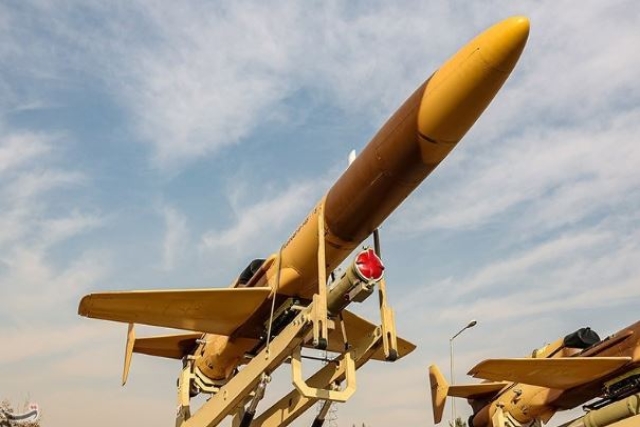The photo captures an upward view of a missile or drone mounted on a yellowish-tan metal launching mechanism. The object, which has a distinct yellow cone at its front, features a wide diagonal brown stripe around its midsection and some lettering just behind the stripe on the yellow part. Extending from the bottom are two short wings, and the back is equipped with steering fins. The mounting piece includes an inverted U-shaped loop that arches over the top of the missile or drone. Notably, at the very end of the launch device, there is a red circle with a red cross, possibly serving as a reflector or light. A similar device is slightly visible off to the bottom right-hand corner of the image. The backdrop consists of a blue sky adorned with wispy white clouds, adding to the clarity of the image taken outdoors.